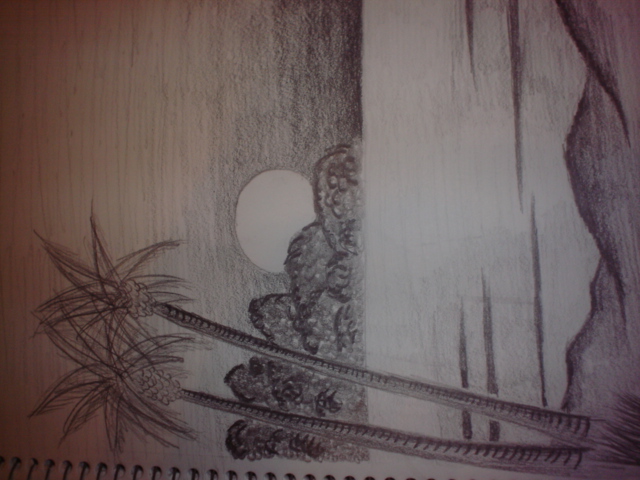This intricately detailed pencil drawing, occupying the majority of a notebook page, is presented rotated 90 degrees counterclockwise. The left edge of the image reveals some black notebook rings. The captivating scene depicts two palm trees standing gracefully on a sandy shore, with patches of grass adorning the foreground. Beyond the serene shoreline lies an expansive body of water, stretching towards a distant piece of land blanketed with lush, bushy trees. These trees are drawn with a circular, voluminous style, distinct from the slender palms in the foreground. A picturesque sunset graces the horizon, its radiant glow partially obscured by the distant vegetation, casting a tranquil ambiance over the entire scene.